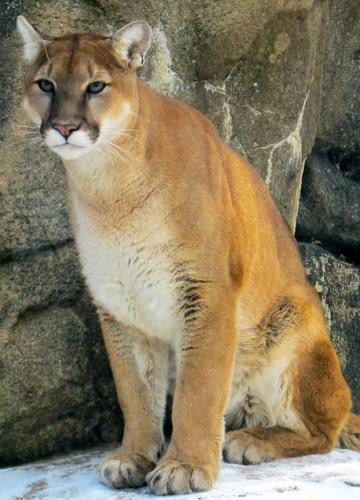This detailed photograph features a close-up of a mountain lion, also known as a cougar, majestically perched on a snowy terrain. The cougar gazes off to the side with its blue-gray eyes, while its perked-up ears and slightly crouched posture reflect alertness and grace. Its striking golden-orange coat contrasts sharply with the snowy white fur covering its chest, belly, and the area around its mouth. The cougar's facial features include darker markings and a slightly gray hue around the face, accentuated by a pink nose and black-outlined snout flanked by prominent whiskers. The creature rests its front paws on the ground, which appears to be a mix of snow and possibly stone. Behind the mountain lion, a rugged rock cliff face, comprised of brown and gray tones with hints of moisture, forms a natural and slightly ominous backdrop. The overall scene suggests a wintery setting in a mountainous wilderness.